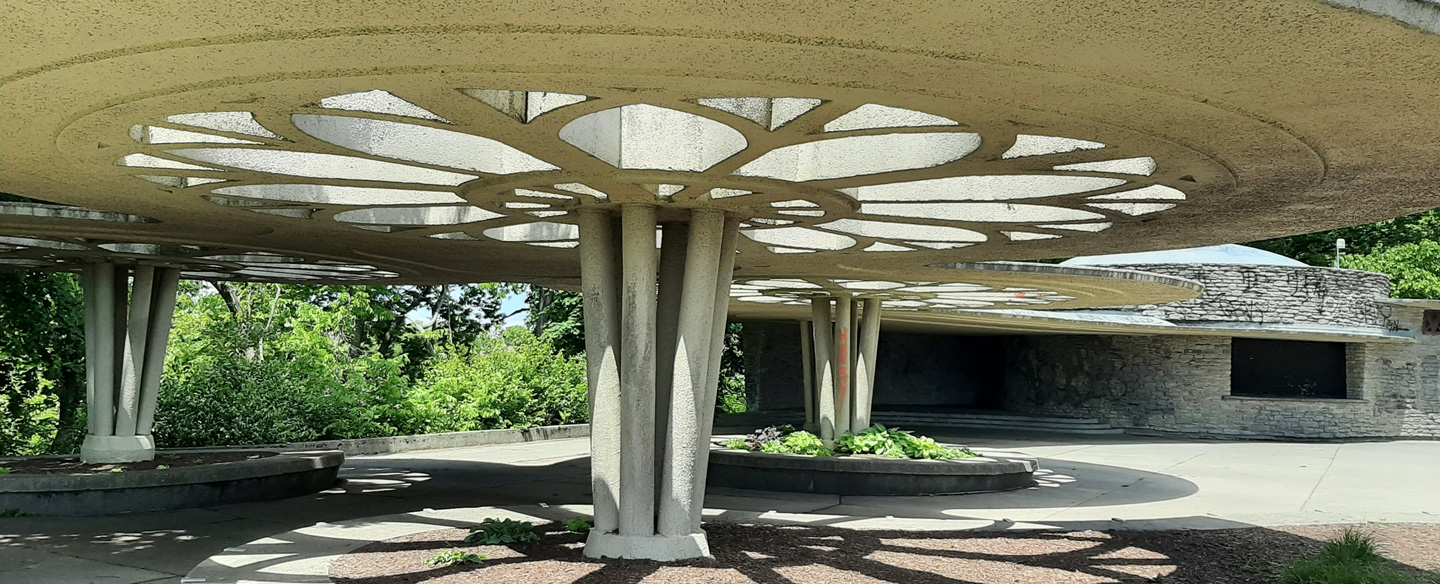In this outdoor photograph, the main focus is a prominent white stone structure with several unique architectural elements. Dominating the scene are three clusters of slender posts, each consisting of five or six smaller angled poles converging to support a concrete platform overhead. This platform features cut-out shapes, creating an intricate latticework that allows sunlight to filter through, casting decorative shadows below. The setting is enhanced by lush green foliage on the left side and in the background, there's a cinder block building with a windowed opening. The sky is visible, offering a hint of blue, adding a serene ambiance to the scene. The structure and surrounding greenery create a harmonious blend of natural and man-made beauty. An additional cluster of similar pillars can be seen towards the back, further enveloped by thriving plants.